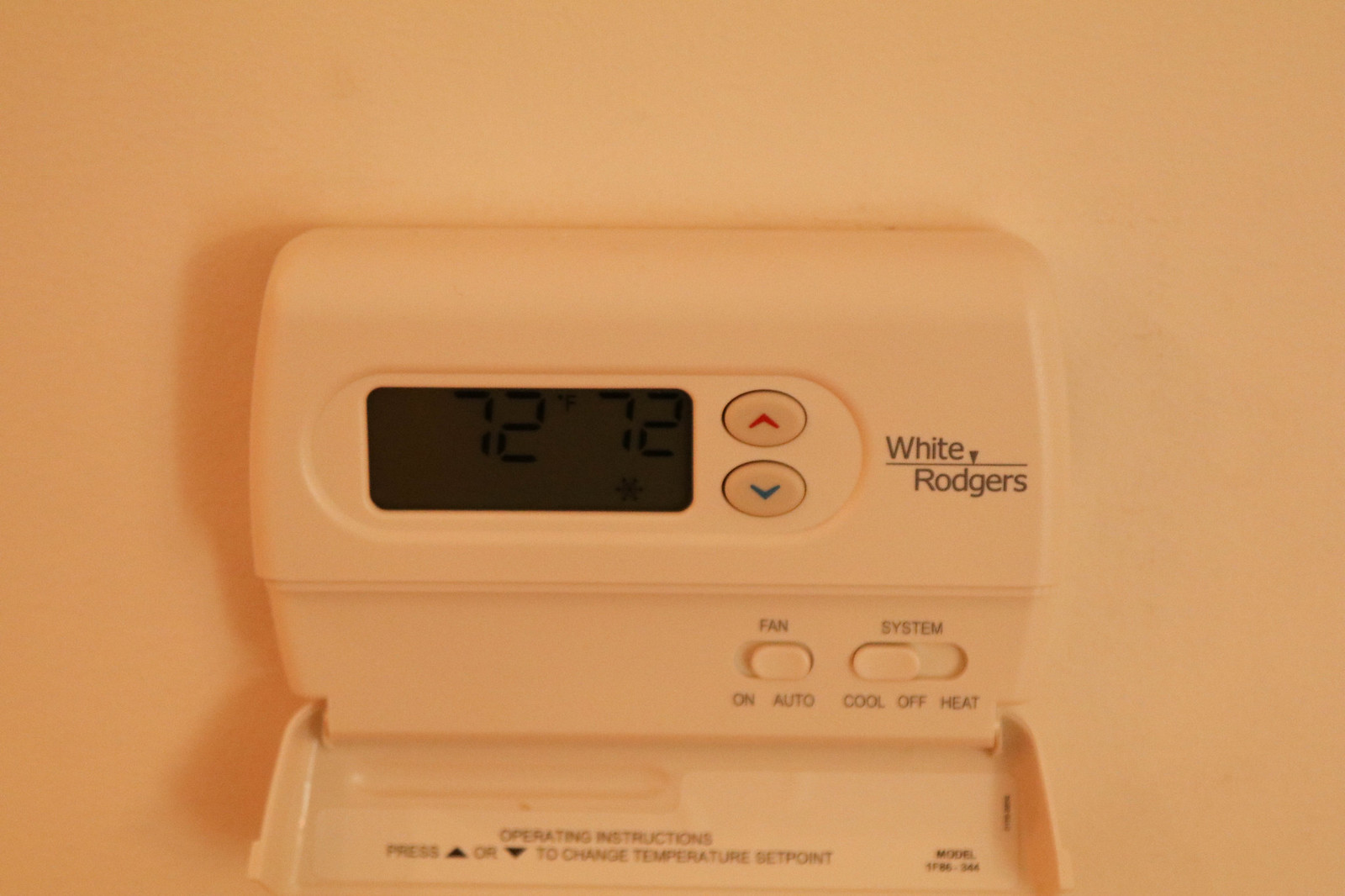A light peach-colored wall serves as the backdrop for a thermostat that blends seamlessly with its surroundings in a similar hue. The thermostat, an oblong box shape, is distinguished by its softly rounded edges and central oval detail. A prominent digital display shows the current temperature of 72.12 degrees. Adjacent to the display are two buttons: one with a red arrow pointing up for increasing the temperature and another with a blue arrow pointing down for decreasing it. Above the display, the name "Rogers" is inscribed in a brown print, underscored by a simple line.

Below the temperature display, there are two long buttons set into a slider configuration. The first button, labeled "Fan," offers options between "On" and "Auto," indicated by brownish-gold print. The second button is for the "System," allowing settings for "Cool," "Off," or "Heat." The front panel of the thermostat is open, revealing the intricate controls beneath. Inside, straightforward directional arrows point up and down, with additional descriptive text aiding in adjustment and setting changes.